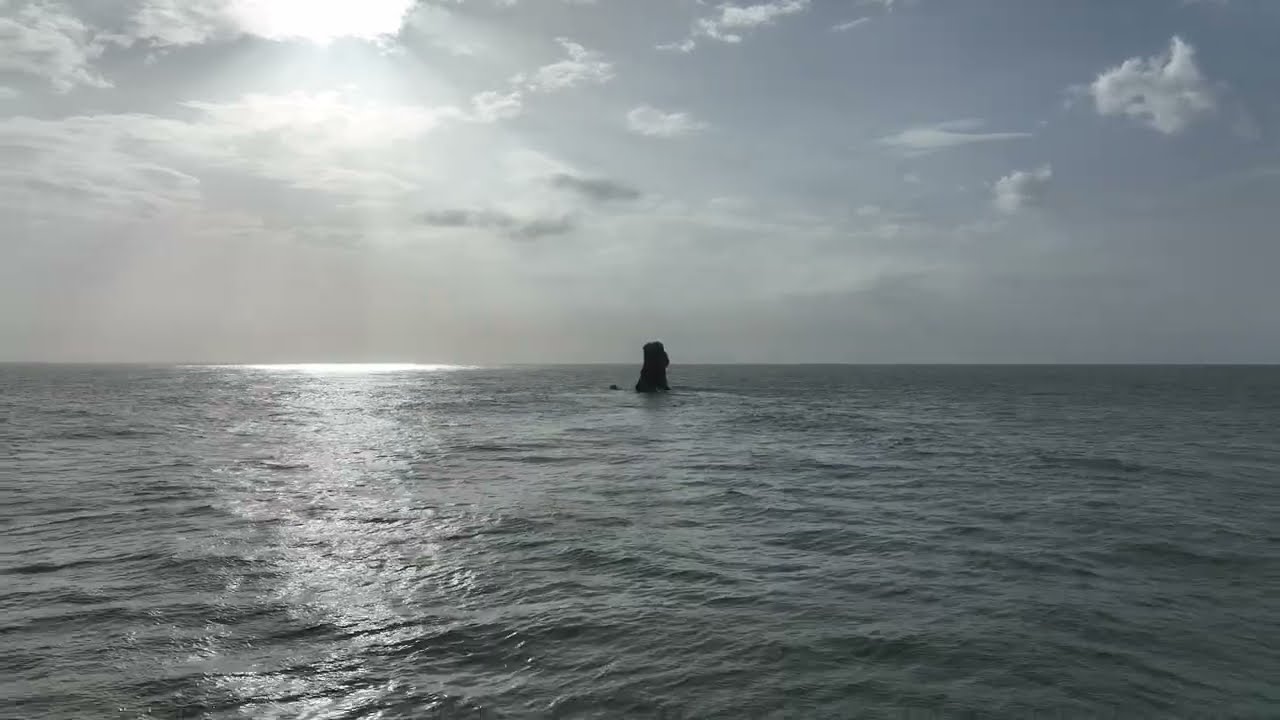The photograph depicts a vast expanse of ocean under a partly cloudy sky. Dominating the center of the image is a small, flat-topped black rock jutting out from the water, creating a focal point that almost resembles a person standing alone amidst the waves. The sky above is a mix of blue and gray tones due to the dense cloud cover, with light seeping through hinting at a bright sun partially obscured by the clouds. Sunlight is creating a bright white spot both in the sky and as a reflection in the clear blue ocean below. The water itself is a deep, dark blue, with mild ripples visible on its surface, adding to the serene yet somewhat gloomy atmosphere of the scene. The overall image is subtly colored, almost monochromatic, which enhances the sense of calm and quietude while capturing the interplay of light and shadow between the sky and the sea.